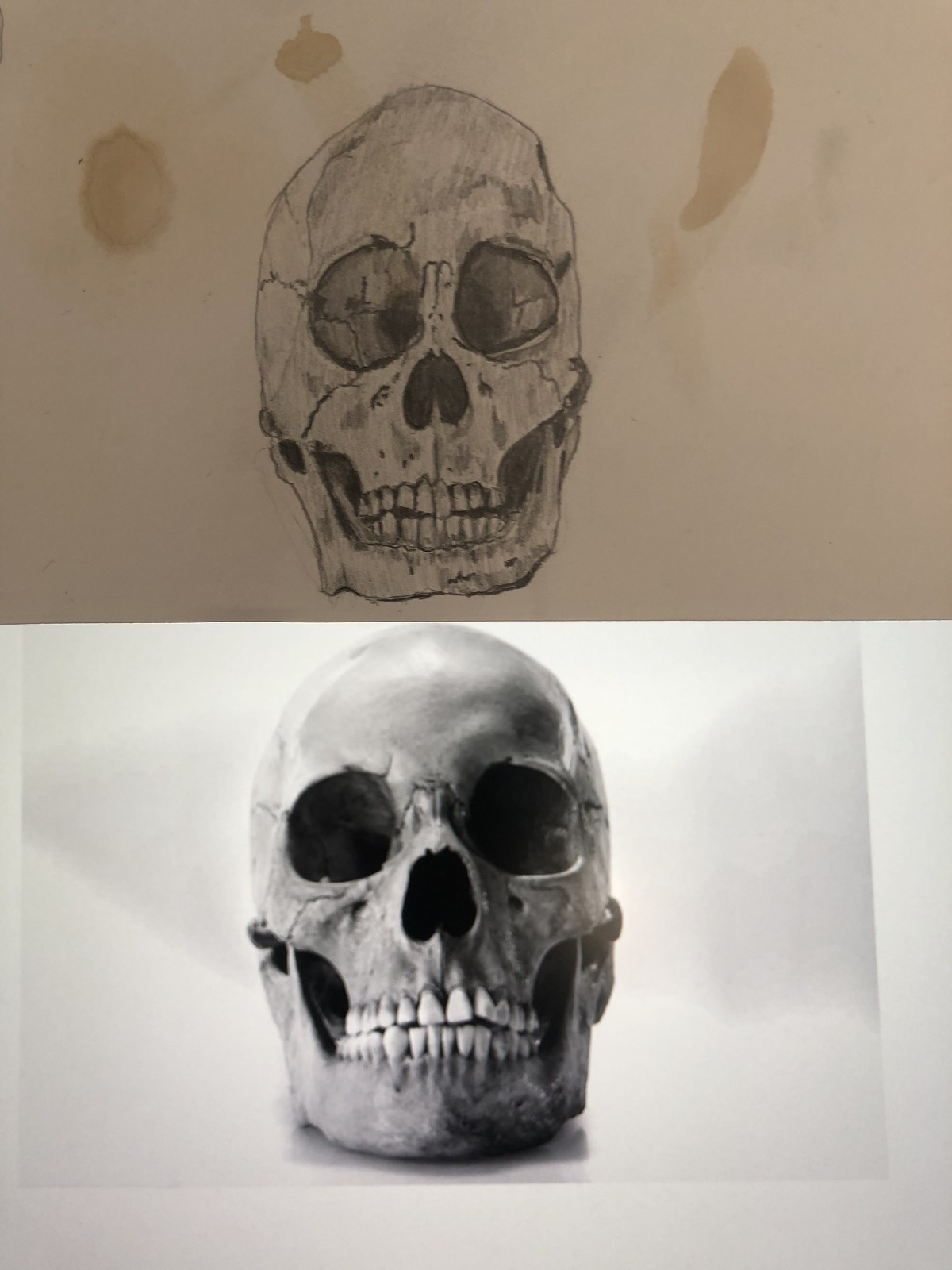The diptych consists of two juxtaposed images, each centering on a skull, positioned one above the other. The upper image, with its brown sepia tint, resembles a hand-drawn or painted artwork on a two-dimensional medium such as paper. The human skull is slightly left of center, showcasing detailed anatomical features including large eye sockets, nasal cavity, jaw, and teeth. Surrounding the skull are several brown splotches — two on the left, one on the right — along with various smudges, possibly created with watercolors or indicative of other staining techniques.

The lower image mirrors the same skull, though potentially slightly larger and situated similarly within the frame. This depiction appears as a lifelike three-dimensional rendering, possibly a digital model or photograph of an actual skull. Set against a clean, white background reminiscent of a mat, it suggests a professional presentation akin to a photographic print or a piece of meticulously curated art. The overall composition invites viewers to juxtapose the intricacies of hand-crafted art with precise digital or photographic realism.